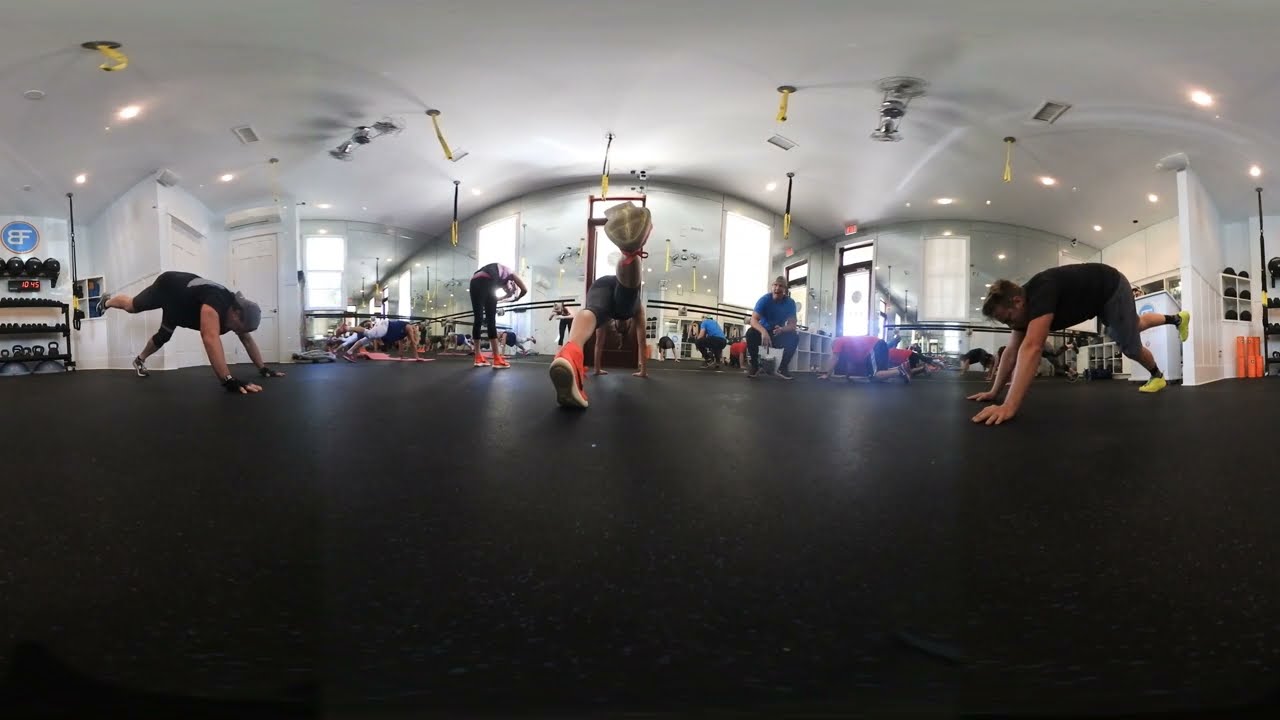The image depicts a large fitness room, possibly in a gym or Pilates studio, with a sleek black rubber floor resembling a yoga mat. The room has white walls and ceiling, accented by yellow bars hanging from above. A prominent blue circle with the letters "EF" is visible, suggesting a fitness-related setting. A mirrored wall reflects the activity in the space.

Approximately ten people are in the room, engaged in various exercises such as stretches and push-ups, all wearing workout outfits that include black short-sleeved shirts, shorts, capris, and leggings. Many sport brightly colored shoes in orange, yellow, or red. 

Centrally located is an instructor in a blue shirt and dark pants, squatting and seemingly giving directions to the group. The 360-degree wide-angle lens captures an expansive view of the room, giving it a slightly distorted perspective that emphasizes the floor while showcasing the energetic activity of the participants.